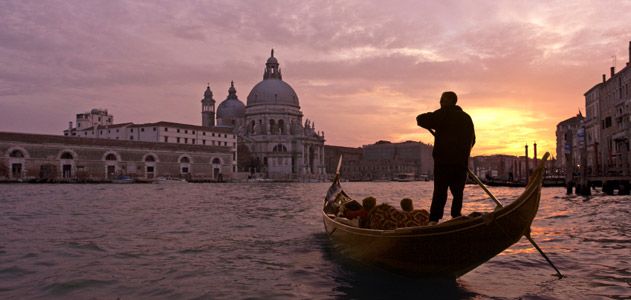This is a photorealistic image depicting a serene evening in Venice, with a richly colored sky in shades of lavender, pink, and yellow, indicating a sunset partially obscured by clouds. Dominating the foreground is a classic Venetian gondola, where a person is seen lying down while another stands, guiding the boat with a gondola pole. The standing gondolier is shrouded in shadow, his features obscured by the dim light. The water stretches out into the mid-ground, reflecting the soft hues of the sunset. In the distance, elegant Venetian buildings reach down to meet the water. Central among them, a magnificent Catholic cathedral stands with its prominent twin domes and a towering spire, accompanied by additional buildings to the right. The scene is bathed in a gentle purple filter, enhancing the tranquil and picturesque atmosphere of this iconic cityscape.